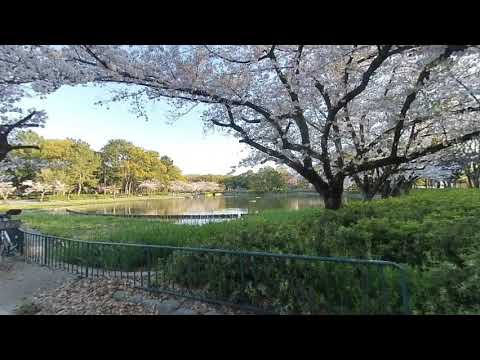The photograph captures a serene scene within a park on a sunny day. Dominated by a strikingly large tree on the right side, adorned with white blossoms, the area is enclosed by a low black metal gate and lush green shrubbery, some of which are bordered by metal gratings. Beyond the gate, a paved pathway scattered with dried leaves meanders through the landscape. The centerpiece of the scene is a calm, almost ripple-free lake with greenish waters that reflect the surrounding nature. Flanking the lake are rows of trees, some bearing white blossoms and others heavy with vibrant green leaves. The background features additional green trees and a slight hill under a mostly blue sky dashed with a few white clouds, creating a picturesque and tranquil park atmosphere.